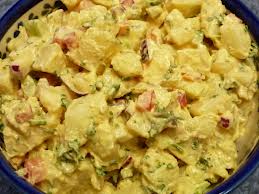The image depicts a close-up of a large bowl filled with creamy tortellini pasta, featuring elements consistent with other descriptive elements of potato or egg salad. The bowl, partially visible, has a dark blue rim with white and floral designs on the interior. The contents of the bowl feature tortellini pasta mixed with colorful vegetables such as red tomatoes and green veggies, possibly onions, all enveloped in a thick, yellowish, cheese-like sauce. The bowl's fullness limits visibility of other details, but the composition rests on a grey countertop. The pasta and vegetables are well-coated, indicating a richly textured dish within the decorative confines of the bowl.